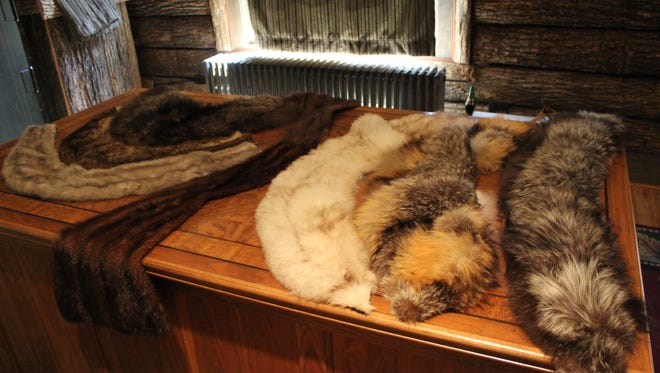The image showcases a rustic, indoor setting featuring various animal furs laid out on a medium-colored wooden table with distinct grain and texture. Behind the table, a wood-paneled wall stands alongside what appears to be a radiator beneath a window with closed curtains. On the left side of the table, three fur stoles or collars are arranged in a curved, overlapping manner; the closest is white, followed by a medium-toned pelt, and the darkest one next to the wall. A long, draped scarf-like fur hangs off the edge of the table. On the right, three more pieces are visible: one white, one brown-gray, and a black and white one. The furs, possibly from various animals, add a natural, somewhat workshop-like ambiance to the scene. The overall color palette includes various shades of brown, white, off-white, some off-reds, and hints of orange, reflecting a nature-inspired, rustic aesthetic.